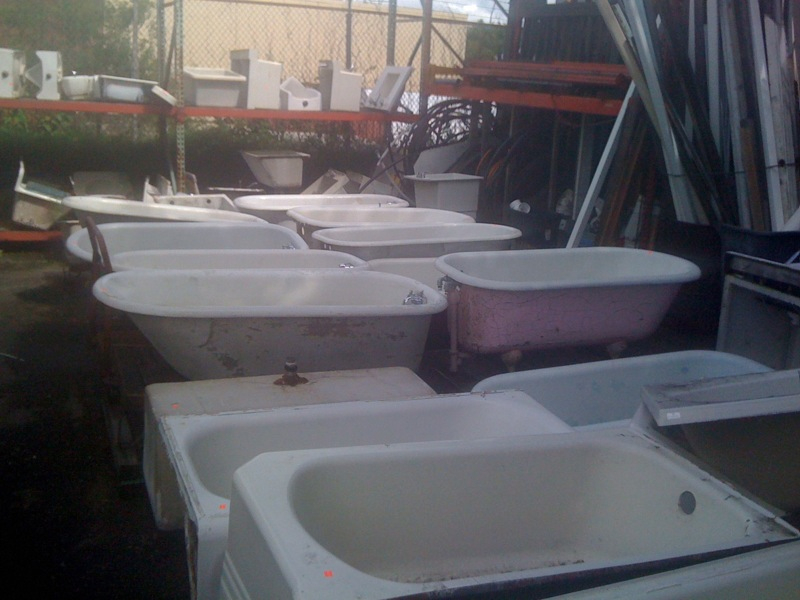The image depicts an outdoor storage yard, likely part of a recycled or vintage bath retailer located within an industrial park. The yard is densely filled with a diverse assortment of used bathtubs in various shapes, sizes, and colors, including a noticeable baby pink tub amidst more subdued dark browns and blues. Two prominent rows of these bathtubs occupy the foreground, each featuring different fixtures like rounded sides or distinctive feet. Surrounding this central area, redwood-colored shelving units hold additional bathroom items such as square Belfast sinks and toilets. To the right, barrels contain tall, thin items like pipes or guttering. The entire yard is enclosed by a high fence, and a large warehouse wall is visible in the background, suggesting this is a commercial establishment repurposing salvaged bathroom fixtures.